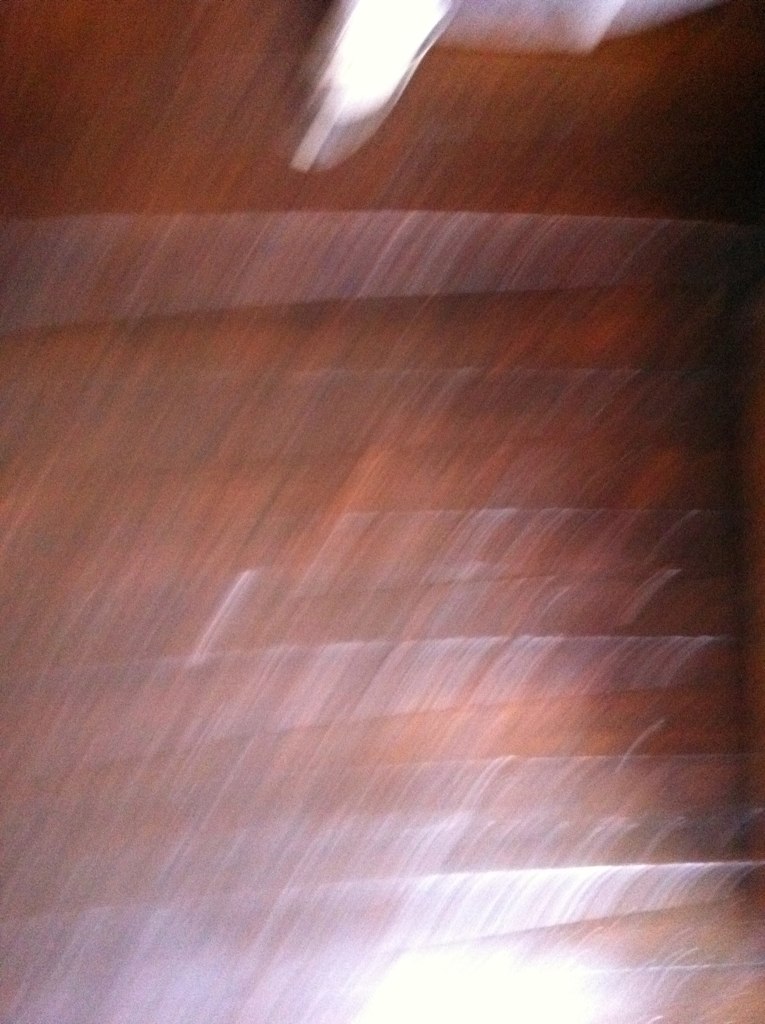A highly blurred photograph featuring severe light glare and a shaken camera effect, making clear identification challenging. The image predominantly shows a reddish-brown surface, possibly part of a wall, although the details are obscured. At the top, an indistinct, oval-shaped white object is vaguely visible. The image is marred by significant white and off-white streaks running vertically, with additional red streaks adding to the distortion. The poor lighting and overall blurriness render the photograph nearly indecipherable.